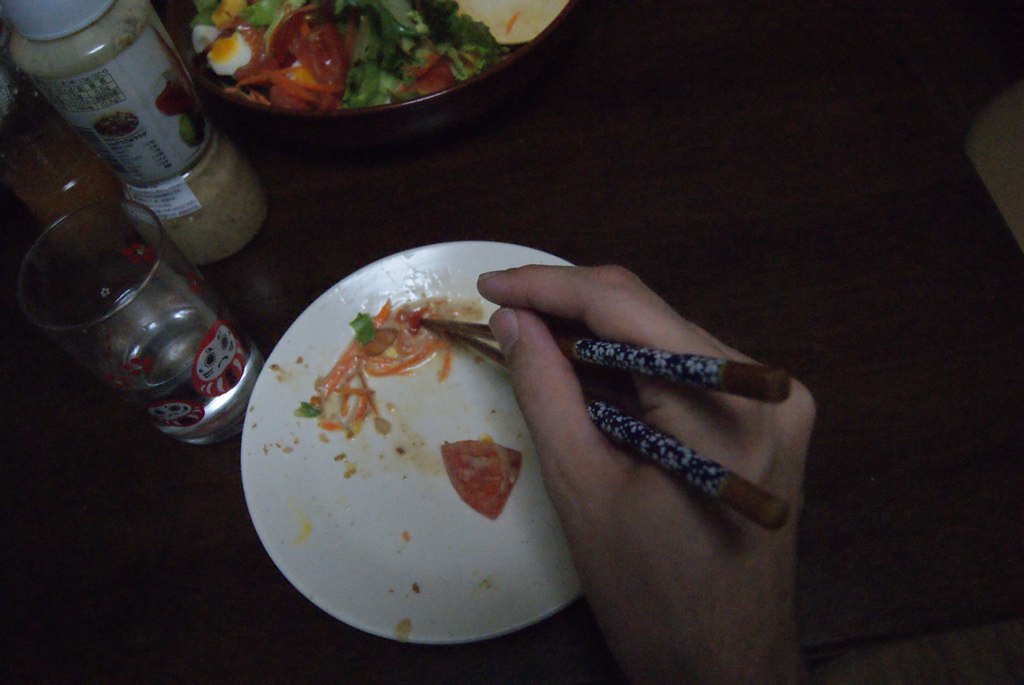The photograph captures an intimate dining scene featuring a light-skinned hand holding dark wooden chopsticks with a white and blue speckled wrapping around the handles. The chopsticks are poised over a nearly empty white plate, grasping at tiny remnants of food, including julienne carrots, a small piece of tomato, and bits of lettuce, possibly from a salad. The plate rests on a dark brown wooden table. In the background, there is a large brown bowl brimming with a fresh salad that includes green lettuce, red tomatoes, carrot slices, and egg pieces. To the left of the plate, a clear glass with water, about a third full, and a tan bottle of sesame sauce are also visible, adding to the detailed and vivid portrayal of someone's mealtime.